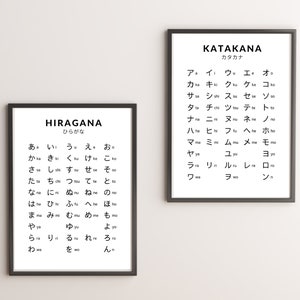The image features two framed posters hanging staggered on a pristine white wall. Both posters are styled in black and white, showcasing the Hiragana and Katakana alphabets of the Japanese language. Each poster is bordered by a sleek black frame. The left poster is titled "Hiragana" in Romaji and also displays the title in Hiragana script, followed by the full Hiragana alphabet. The right poster, positioned slightly above and to the right, is titled "Katakana" in Romaji and Katakana script, accompanied by the complete Katakana alphabet. Both alphabets are organized in vertical lines, encompassing sounds like A, E, I, O, U, and combinations such as MA, ME, MI, MO, MU, and BA, BE, BI, BO, BU. This detailed presentation exemplifies the core elements of Hiragana and Katakana, integral components of the Japanese writing system.